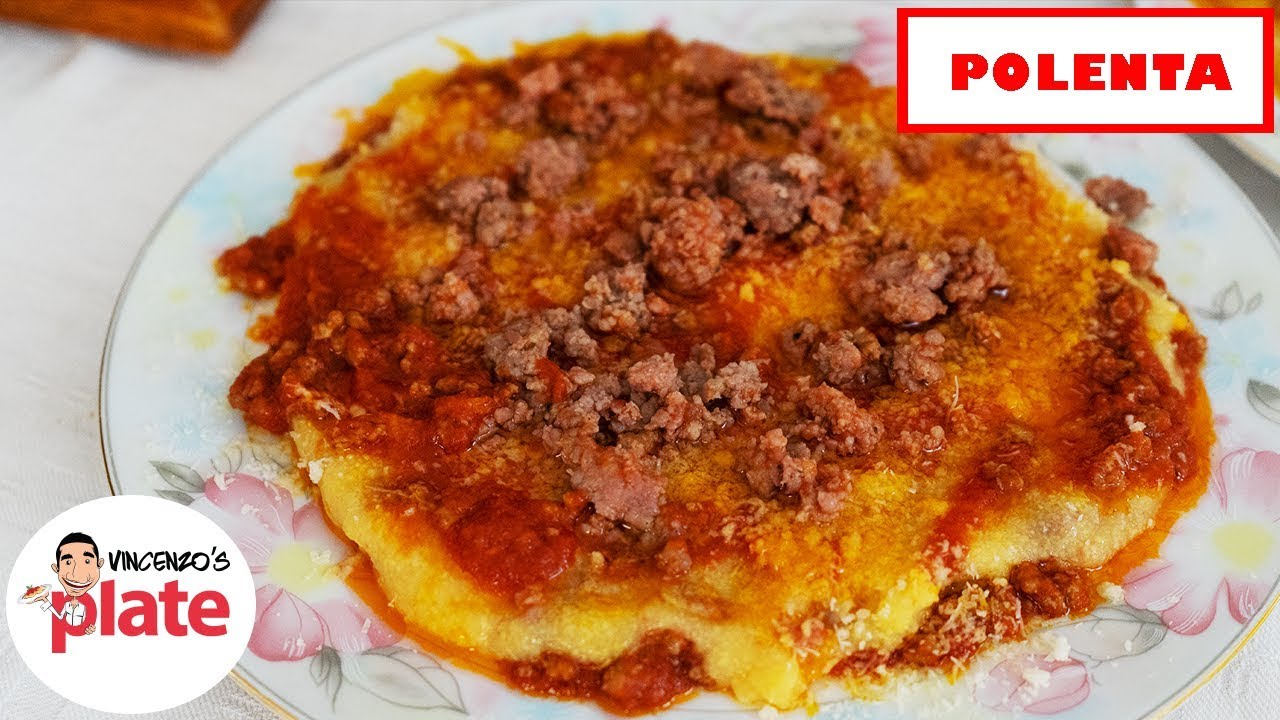This photograph captures a vibrant dish of baked polenta served on a white porcelain plate adorned with pink flowers and green leaves around the rim. The centerpiece polenta is topped with a rich red sauce and scattered pieces of hamburger meat. A layer of browned crust on the top suggests it has been oven-baked to perfection, making it look heated and ready to eat. Additional garnishing includes shredded white cheese sprinkled over the top. On the top right corner of the image, "polenta" is written in bold red letters inside a red rectangular border, while the bottom left corner features a logo that reads "Vincenzo's Plate," accompanied by a drawing of Vincenzo holding a plate of food resembling the one in the photograph. This detailed and colorful image appears to be an advertisement for Vincenzo's Plate, inviting viewers to savor this hearty and appetizing dish.